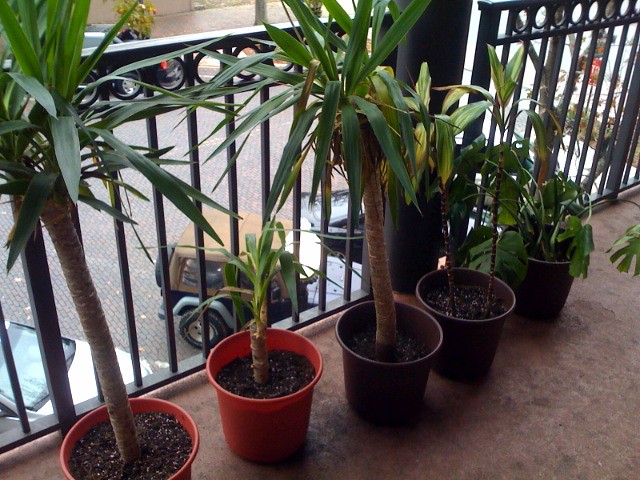The image portrays a slightly wider-than-tall view from normal person height, looking down on a second-story balcony or porch with a distinctive brownish-red stone or stucco floor. There are five flower pots neatly arranged along the edge of the balcony, bordered by a black wrought iron fence. The first two pots are medium red in color, the next two are brown, and the last one is black. The first three pots contain young palm trees; the first two are particularly tall, while the third is much shorter. The fourth pot appears empty or the plant is not visible, and the fifth pot contains a plant with long leaves in close proximity to the pot, resembling a vine. Below the balcony, a street can be seen with several parked cars, including a Jeep, two sedans, and others across the street, on what looks like a brick or cobblestone road. The overall perspective and angle suggest that the photo was taken with a phone camera.